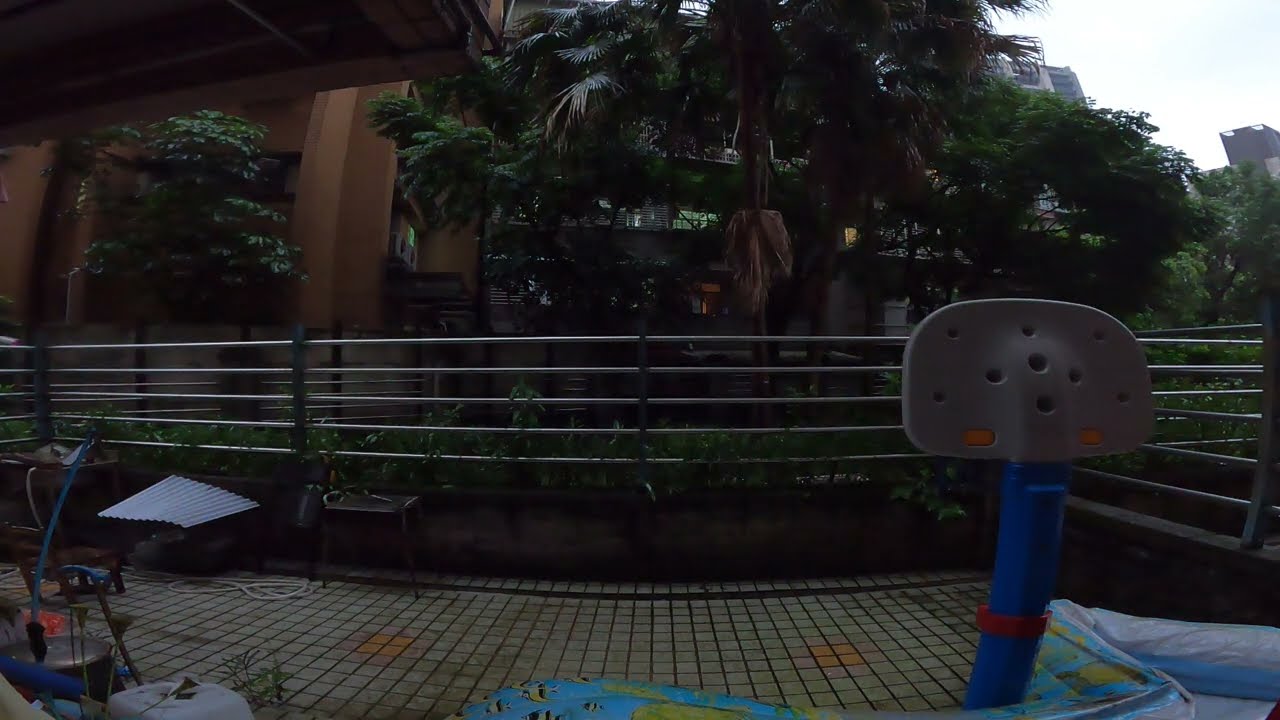In this outdoor photograph of a back patio in an elevated apartment building, we see an enclosed space surrounded by a tall metal railing and covered in what looks like tile flooring. The scene is cluttered with various items scattered on the slightly dirty ground, including toys and what appears to be a plastic kid’s basketball hoop in the bottom right corner. A blue and gray shovel-like object is sticking up, though its exact function is unclear. Amidst the messiness, green vegetation is thriving, with palm trees and other types of green shrubs and bushes visible around the patio. Beyond the railing, the background reveals more apartment buildings and balconies, partially obscured by the lush tropical foliage. The sky above is overcast, casting a diffused light over the scene, suggesting it is in the middle of the day. There are no people present in the image.